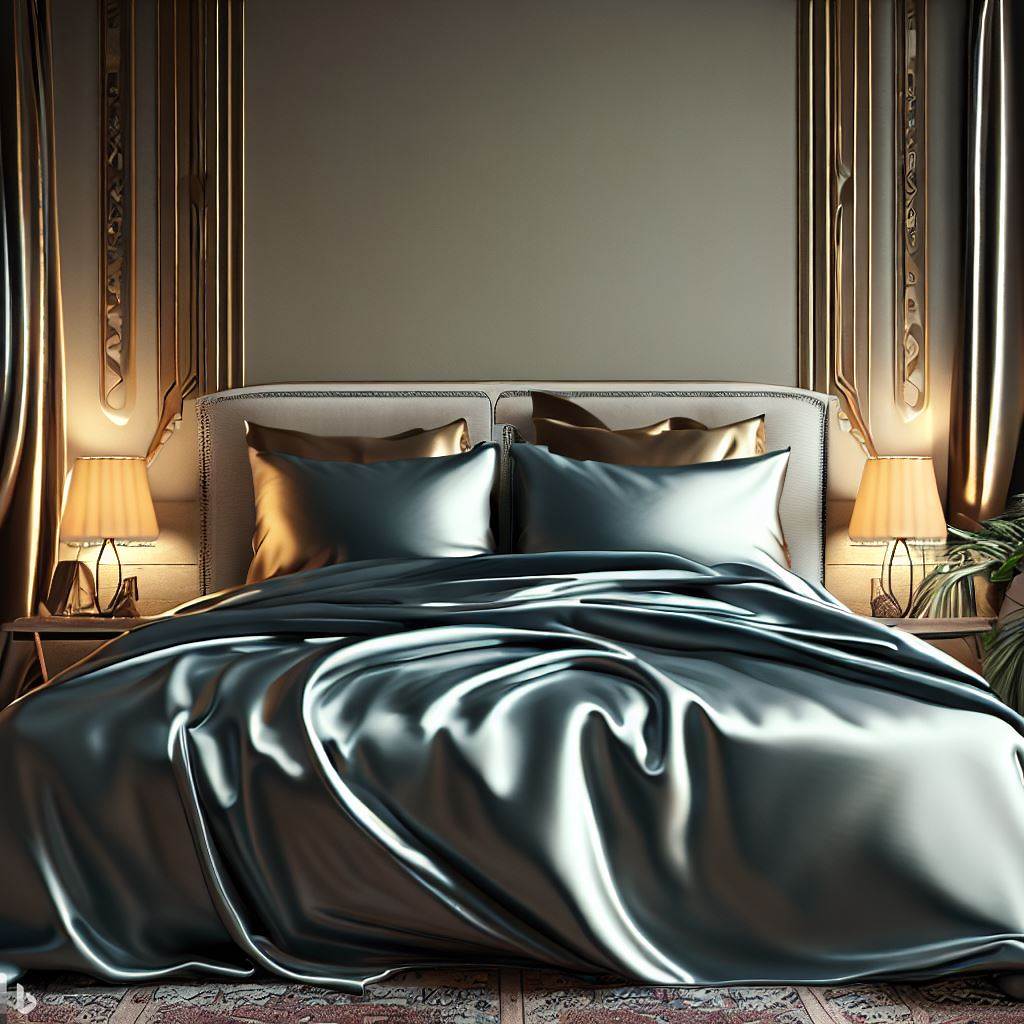The photograph captures a lavish and luxurious bedroom, centered around a grand bed adorned with a grey-silver velvet or possibly satin comforter. At the forefront of the bed are two pillows matching the grey-silver color of the bedding, while behind them lie two golden pillows, adding a touch of opulence. The bed is anchored by a padded headboard that appears to be crafted from grey linen or a beige-silver material, providing a sophisticated backdrop.

On each side of the bed, nightstands hold identical lit lamps, casting a soft glow that enhances the room's warm, metallic ambiance. To the right, a potted plant's branches partially emerge into view, adding a natural element. The walls feature intricate bronze floral designs in the upper corners, further accentuating the room's ornate decor.

The focus of the image is undoubtedly the bed, draped in luxurious fabric and meticulously styled to emphasize its elegance—an impression that suggests the room could be part of a high-end hotel or an advertisement for a bedding set. The overall color palette is dominated by rich metallics, mainly golds and silvers, enhancing the room's lavish aesthetic. A small, lowercase 'b' watermark is visible at the bottom right corner, with no other text or people present in the photograph.